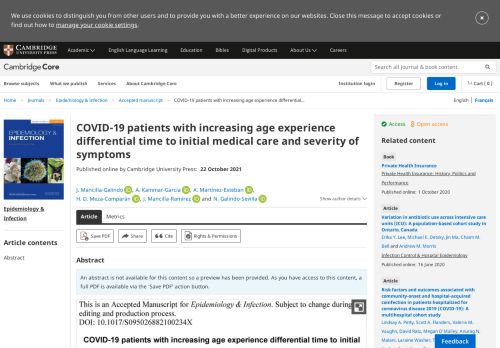The image displays a webpage with a gray header at the top that informs users about the use of cookies to provide a better experience and offers options to either close the message or manage cookie settings. The header identifies the website as "Cambridge Core." Below the header, the page contains several navigation options, though they are too blurry to read clearly. 

Prominently featured on the page is a blue square labeled "Infection," with the main text highlighting research on COVID-19. It states, "COVID-19 patients with increasing age experience differential time to initial medical care and severity of symptoms," and notes that the article was published online by Cambridge University on October 22, 2021. 

Further down, there is an "Abstract" section enclosed in a blue box, explaining that the manuscript is accepted for publication in "Epidemiology and Infection" but is still subject to changes during the editing and production process. The abstract reiterates that older COVID-19 patients tend to experience delays in seeking initial medical care as well as more severe symptoms.